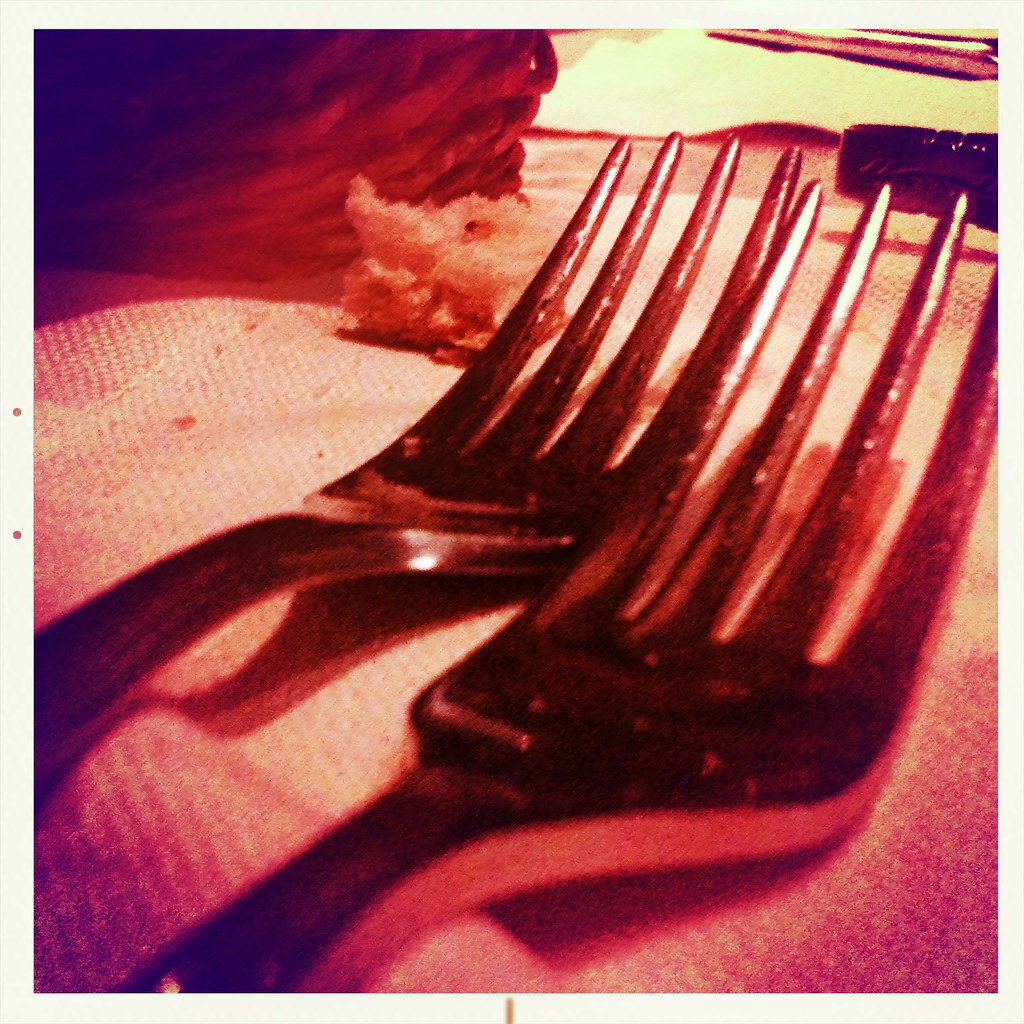The photograph features an up-close view of two forks, a larger dinner fork on the right and a slightly smaller salad fork on the left. Both forks have dark hues with red reflections, indicating they may have been used, reflecting the ambient light in the scene. They rest on a woven piece of fabric or tablecloth with peach tones and red shadows around the edges. In the background, there are various dinner-related items. To the left, there is a large, brown crumb of food, likely batter from a fried item. Above it, in the top-left corner, a woven basket can be seen, suggesting a breadbasket or similar container. The top right reveals a black cylindrical object lying sideways, next to which is a piece of white paper, possibly napkin. The entire scene is tinted with a high-contrast filter reminiscent of old Polaroid photographs, dominated by red, purple, and yellow tones. This filter gives the image a retro feel, with yellower whites, purpler blacks, and a vignette adding to the nostalgic atmosphere.